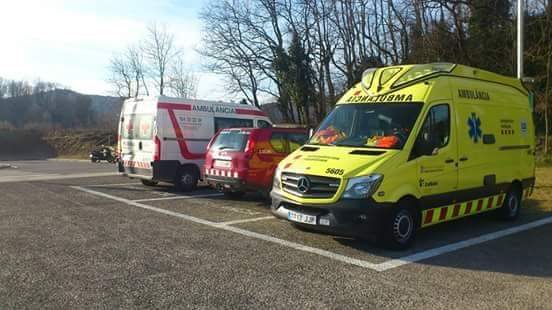The image depicts a parking area, possibly at a hospital or an emergency services location, with three specific parking spaces. In the nearest spot to the front of the photograph, there is a bright yellow ambulance with the Mercedes logo on its grille and bright orange high-visibility items in the windshield, facing left. The middle space is occupied by a small red SUV-like vehicle, presumably a paramedic or emergency services car, identifiable by emergency tape on its rear, with its front pointing to the bottom left of the image. The third space has a white ambulance with red markings and the word "Ambulanza" on it, facing to the right. In the distance, beyond these vehicles, four other vehicles can be seen. To the left of the scene, a building with a hill, and a black car, are also visible. The background also features barren trees, indicating a likely autumn or winter setting, and there is a white post behind the yellow Mercedes ambulance.